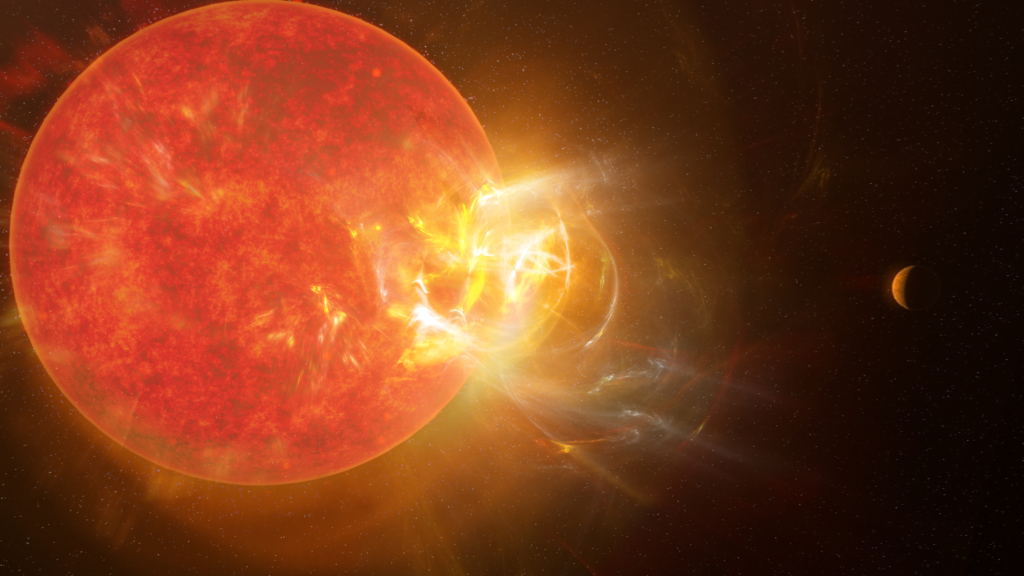The image depicts a vivid digital or AI-generated scene of a colossal star, most likely the Sun, dominating the left side against the stark backdrop of a black sky. The Sun is a striking mix of dark red and bright orange hues, punctuated by patches of yellow, and exhibits a prominent solar flare extending from its fiery surface. This flare is brightly yellow and snakes outward, creating a dynamic sense of energy. Surrounding the Sun is a noticeable yellow halo. To the right, in stark contrast to the Sun's brilliance, lies a much smaller, round, brownish planet, possibly Mercury. The planet is partially illuminated by the Sun, with the left side bathed in light while the right side fades into darkness. The absence of other stars or celestial bodies in the background emphasizes the isolation and stark beauty of this cosmic tableau.